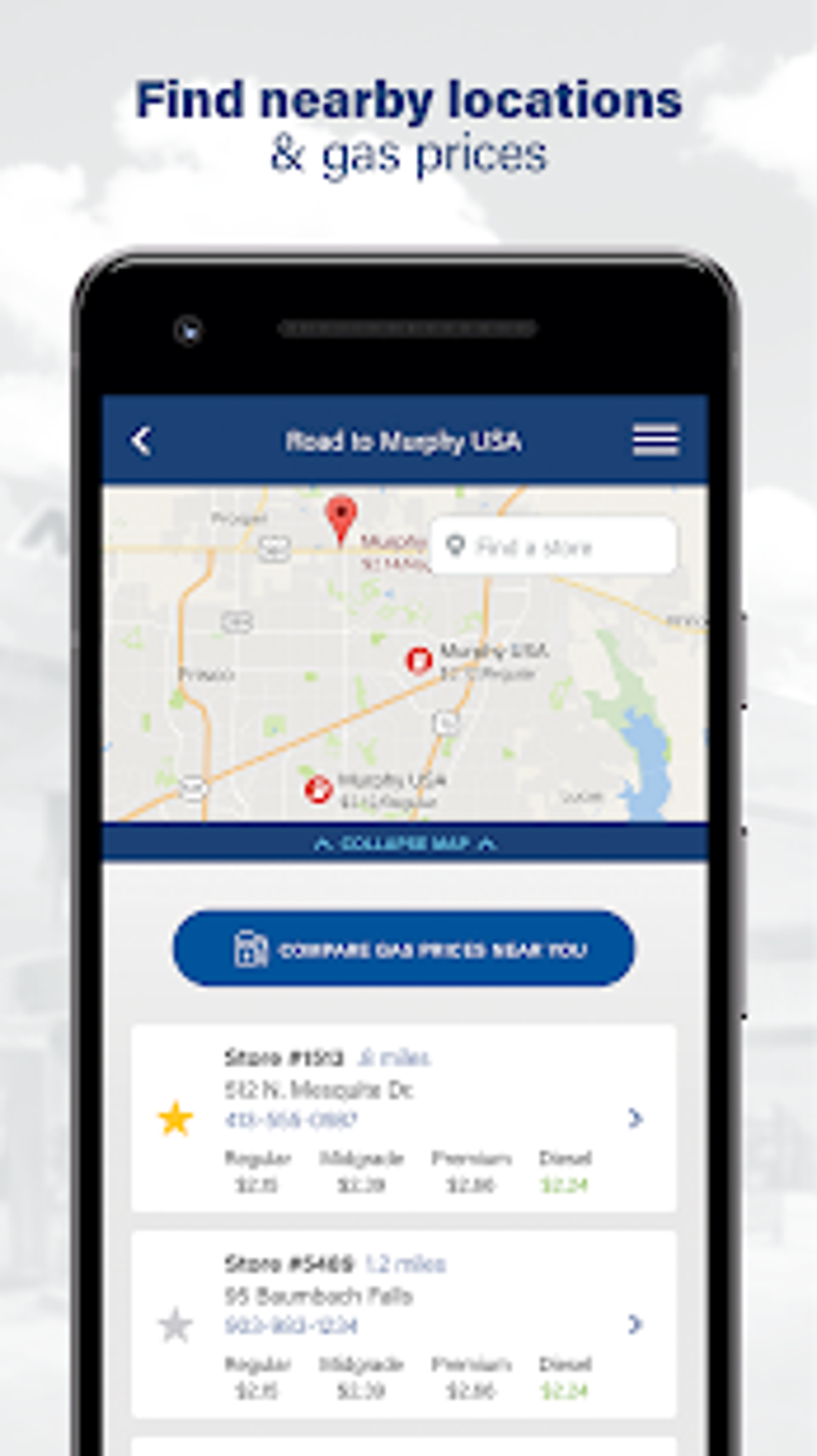A highly pixellated and blurry screenshot of a smartphone mock-up is displayed. The image appears to be significantly enlarged, causing noticeable pixelation. Nonetheless, the outline of the phone is discernible, featuring the edges, side buttons, metal framing, and specular highlights on the curved top of the glass.

Within the smartphone's display, the image showcases a search application interface. At the top of the screen is a blue bar with a header reading "Road to Murphy USA," accompanied by a hamburger menu icon on the right. Below this, the app interface includes a section for Google Maps, labeled "Find Nearby Locations and Gas Prices."

The map displayed in the background shows various details, including a pinned location near the northern side, a road, and a green and blue section indicating the outline of a lake. 

Below the map, a text header reads "Compare Gas Prices Near You." Underneath this header, there are two rectangular sections, each displaying store information and corresponding addresses. Star options for ratings appear to the left, with the top store selected via a gold star. Unfortunately, specific price details are illegible due to the pixelation.

Overall, the image attempts to detail an application designed to help users find and compare gas prices at nearby locations, but legibility is hindered by the poor image quality.